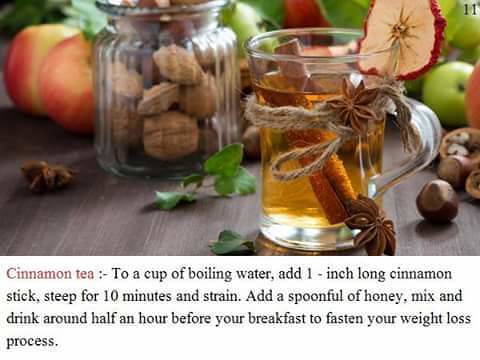This beautifully arranged photograph captures a clear glass cup of cinnamon tea, garnished with a slice of fruit on its rim, resting on a wooden table. The glass cup, adorned with a rustic rope tied around its middle, contains a rich brown liquid with a visible cinnamon stick submerged in it, indicating it is the cinnamon tea mentioned. Surrounding the cup are scattered walnuts and apples, with a jar of uncracked walnuts placed nearby. In the background, additional fruits like apples and possibly peaches are interspersed with some greenery, adding to the natural aesthetic. Below the image, the text in red reads "Cinnamon Tea," followed by the preparation steps in black: To a cup of boiling water, add one-inch-long cinnamon stick, steep for 10 minutes, strain, and then add a spoonful of honey. Stir well and consume approximately thirty minutes before breakfast to enhance your weight loss efforts. The image is not just about the tea but also exudes a sense of homely warmth and natural ingredients, complemented by the numbered "11" in the top right corner, hinting at its sequence in a series.